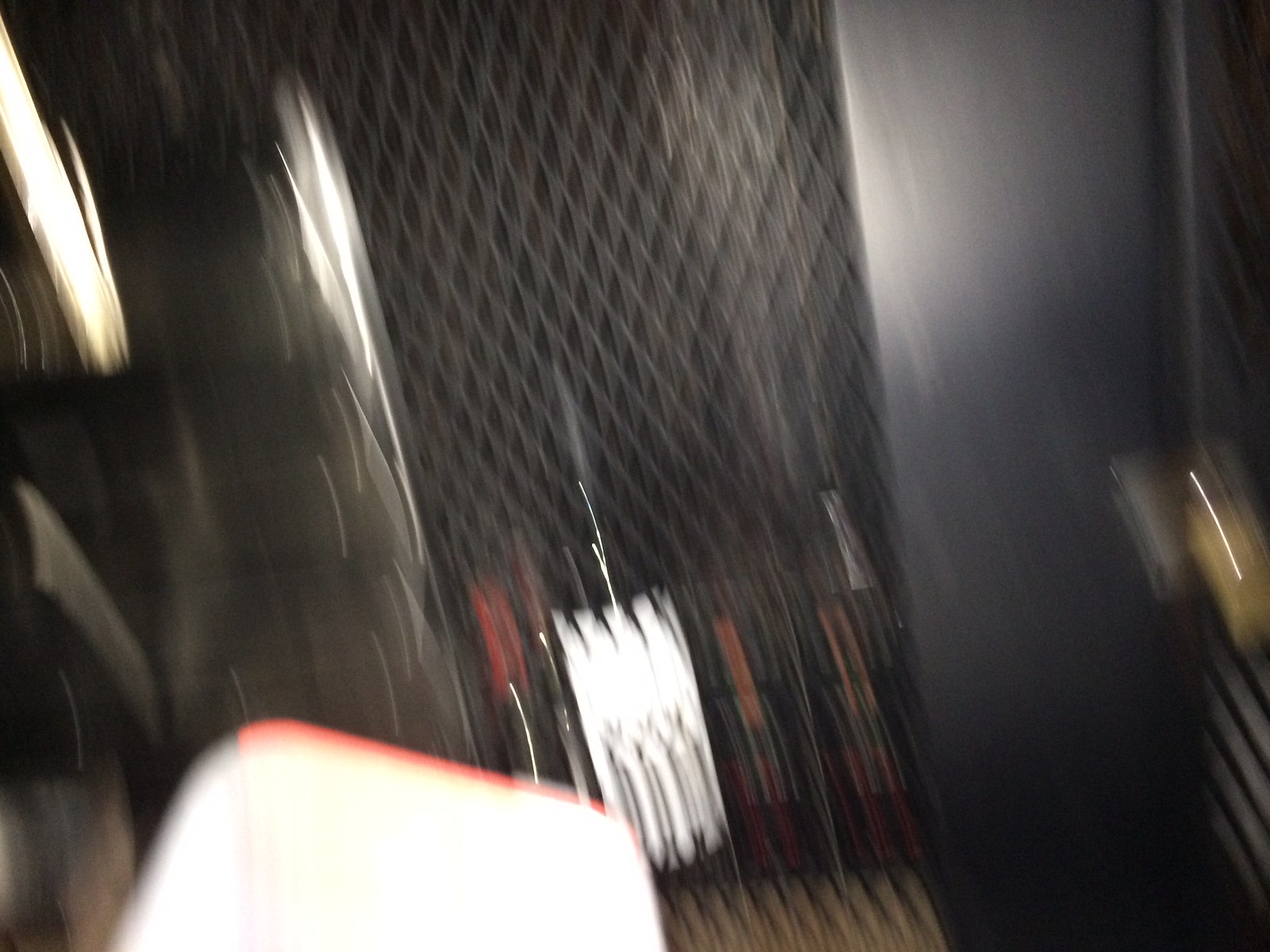This image is heavily blurred, making it challenging to identify specific details clearly. However, it appears to depict the separation between two train cars. There is a metal gate, characteristic of those found between such cars, which typically close off sections once passengers have moved through. Adding to the confusion are entwined white and red wires, elements unusual for a train setting. The dominant metal structure could also suggest an old elevator with a gated entrance. In the lower left corner, there is a white, box-like shape, and on the right side, a slotted door is visible. Additionally, there are pieces of machinery situated on the left side of the image.